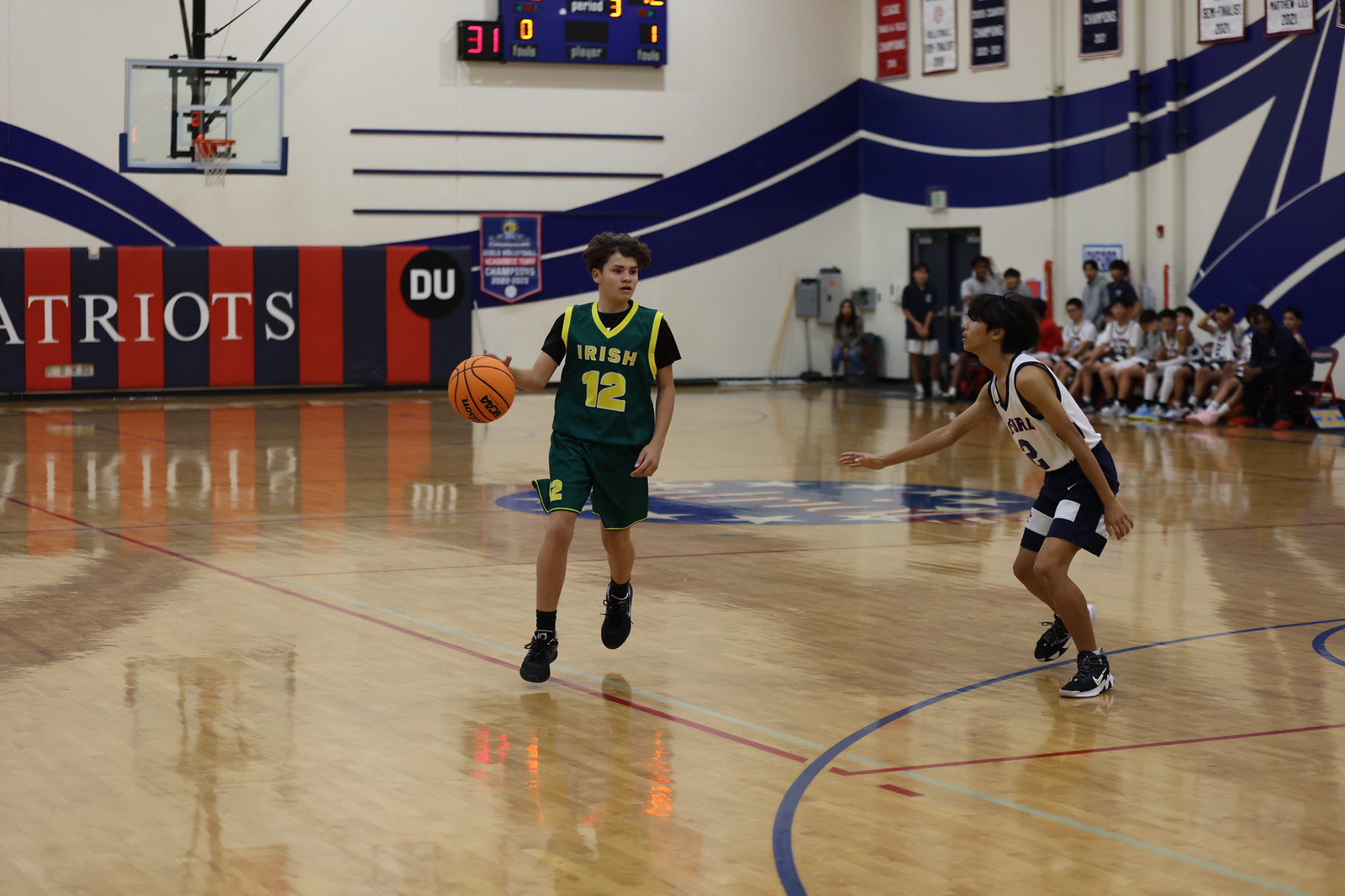The photograph captures an intense basketball game in motion within a gymnasium, featuring teenage boys, approximately 12 to 13 years old. The polished brown wooden floor reflects the action between two players in the foreground. One player, wearing a dark green uniform with yellow lettering that reads "Irish" and sporting the number 12, is dribbling the ball with his right hand. He also wears black tennis shoes, short black socks, and has short black hair. Next to him, attempting to counter, is a player from the opposing team dressed in a white tank top and black shorts, complemented by black and white tennis shoes and white socks. The gymnasium's white walls are adorned with blue line designs, and in the background, spectators are either seated or standing near the boundary, watching the match. On the right side of the photo, other players from the white and black team can be seen sitting on benches. The far back wall features a scoreboard and a basketball hoop, along with a large red and black sign that partially reads "Patriots."